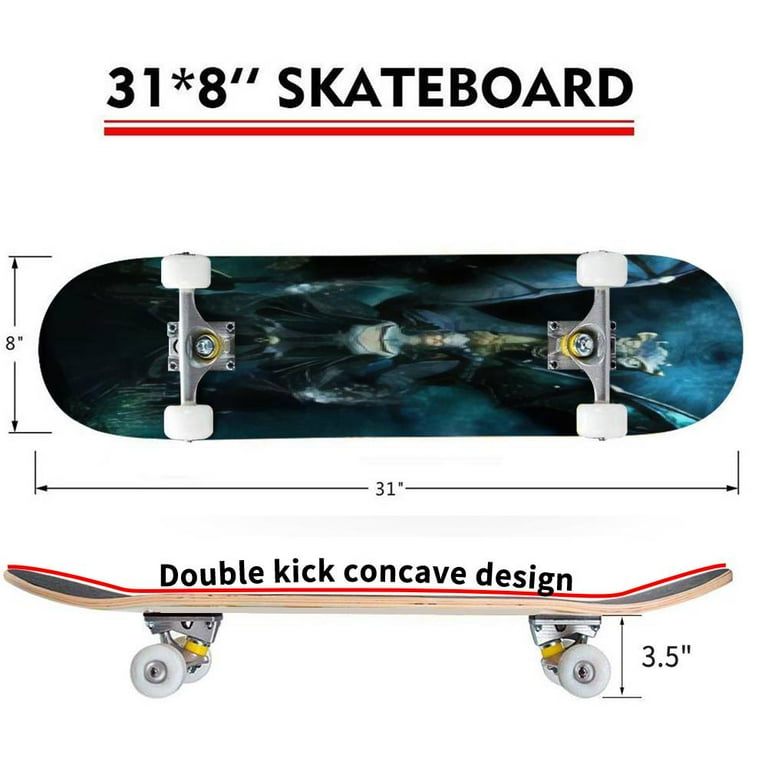The image displays a detailed advertisement of a skateboard, showcasing both the underside and the side view of the board. The skateboard features a dark blue or teal background, adorned with an intricate dragon design, though the exact image is somewhat obscured when viewed horizontally. The skateboard is specified to measure 31 inches in length and 8 inches in width, indicated with the notation "31 * 8 inches." The board includes a double kick concave design, which is visually represented from the side angle. Additionally, the skateboard is noted to be 3.5 inches from the ground to the bottom of the board. The underside of the skateboard, where the dragon design is located, incorporates metallic components and wheels, suggesting it is constructed from wood. Red lines accentuate key features such as the skateboard measurements and the double kick concave design.